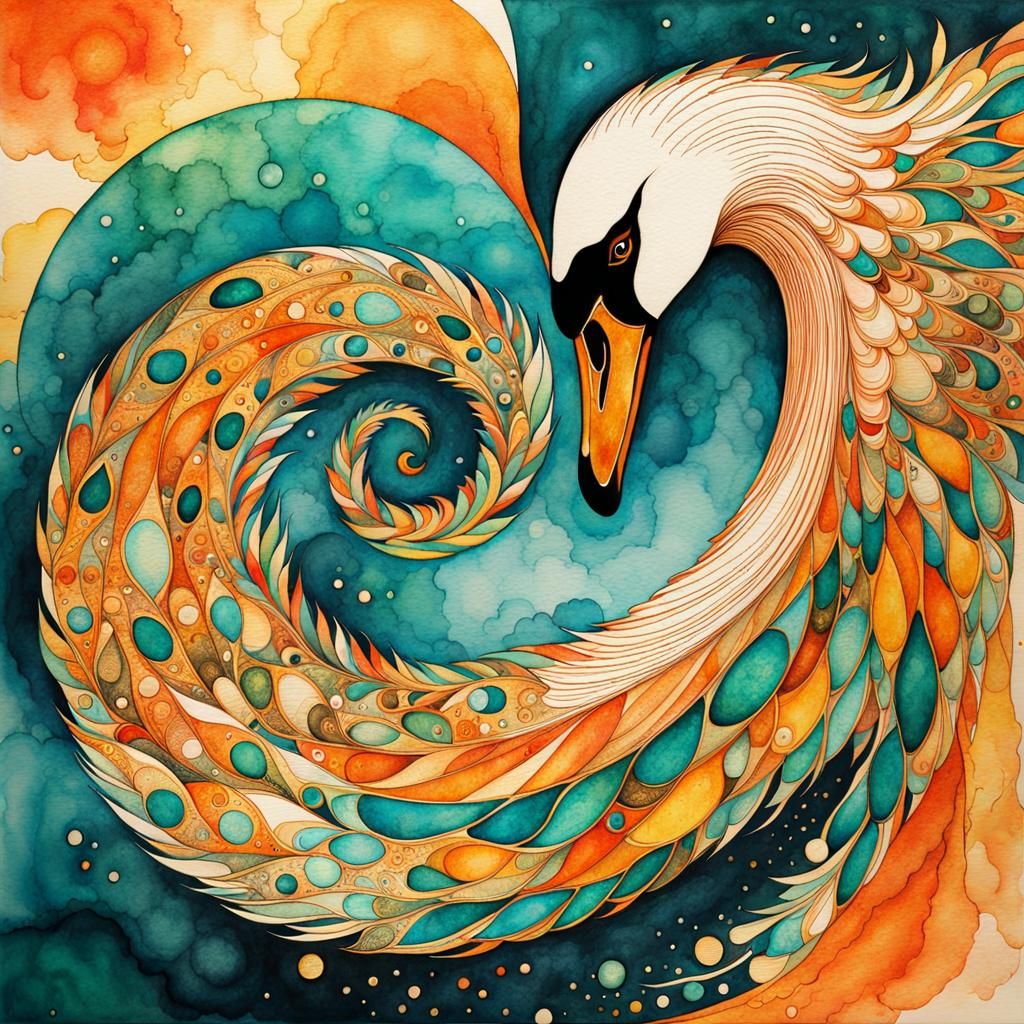The image is a surreal and vibrant watercolor painting depicting a swan. The swan's head, seen on the right side of the composition, features a white head, black markings around the eye, and an orange beak. As the neck gracefully descends, the form transforms into an abstract, continuous swirl, interweaving through the composition and giving the illusion of motion. The swan's feathers display a stunning array of colors, primarily coral and teal, blended in a mesmerizing yin and yang pattern. The background is adorned with swirling teal clouds, dotted with intermittent stars, and interspersed with coral clouds, enhancing the painting's dreamlike quality. The body of the swan circulates in a clockwise pattern, creating a dynamic, circular design that is rich in shades of orange, blue, and turquoise. The overall atmosphere of the painting is both artistic and abstract, celebrating fluidity and color in a compelling visual narrative.